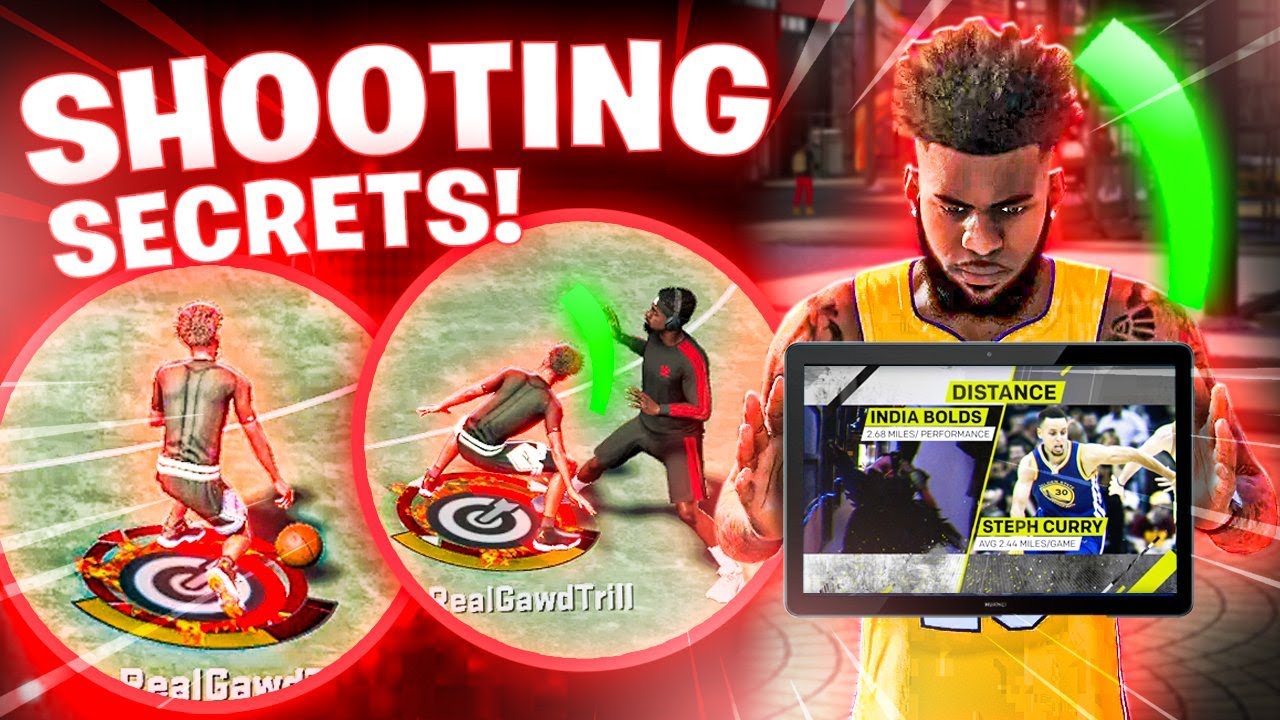The image appears to pertain to a football game and includes several detailed elements. At the top, there is a heading that reads "Shooting Secrets." Below the heading are two red, circular inset images that resemble thumbnail prints, each depicting a man standing within a circular target area. In one of these thumbnails, a football is visible approaching the man, while in the other, the ball is not visible.

Additionally, the central figure in the image is a person with very fuzzy hair, a moustache, and a slight goatee beard. This person is dressed in a yellow tabard worn over a multicolored t-shirt. They are holding a tablet screen which displays two separate photos related to football. One photo has a caption that reads "Stephen Curry," depicting a player in a blue and white striped uniform chasing a ball down the pitch. The other photo is labeled "India Bolds," but its contents are indistinct. The overall composition of the image suggests a focus on football techniques and secrets, with a particular emphasis on shooting skills.